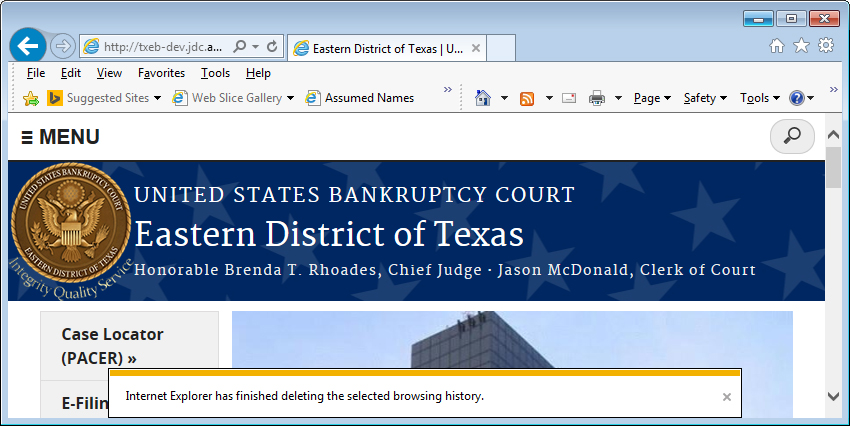The image captures a screenshot from a computer screen, focusing on a tab titled "Eastern District of Texas / U.S. Bankruptcy Court." At the top of the browser window, several menu options are visible, including "File," "Edit," "View," "Favorite," "Tools," and "Help." Below these, there are clickable areas labeled "Suggested Sites," "Web Slice Gallery," and "Assumed Names." The browser window is adorned with various icons, and a distinct menu indicator with three horizontal lines is present.

Dominating the central part of the screen is an emblem of the United States, featuring a golden brown eagle. Below this emblem, the text reads "United States Bankruptcy Court" followed by "Eastern District of Texas." The court's motto, "Integrity, Quality, Service," is prominently displayed. The article on the screen discusses the United States Bankruptcy Court for the Eastern District of Texas, mentioning "Honorable Brenda T. Rhodes, Chief Judge," and "Jason McDonald, Clerk of Court."

Towards the bottom of the screen, a notification from Internet Explorer indicates that "Internet Explorer has finished deleting the selected browsing history," though part of this message is cut off.